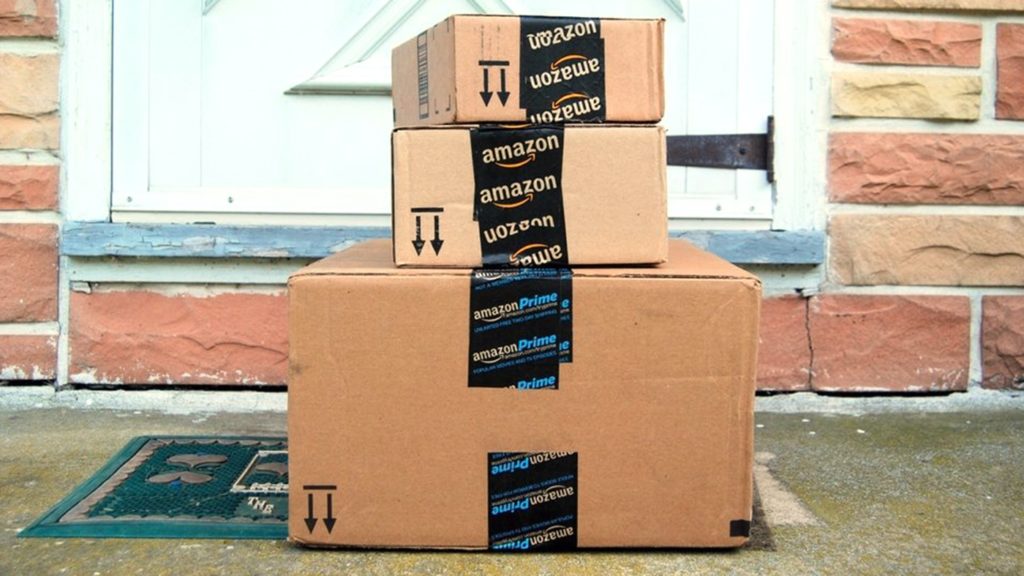Three Amazon Prime boxes are stacked on a doormat in front of a white, wooden doorway of a red brick house. The boxes are arranged with a large one at the bottom, a medium one in the middle, and a smaller one on top, all in descending size. Notably, the boxes are upside down, with the arrows pointing downward. They are brown in color and sealed with black Amazon tape that features white lettering and a splash of blue for the word "Prime." The scene is set on a sunny day, with the well-lit porch showcasing a combination of earthy browns and reds from the bricks, complemented by the clean, white doorway.